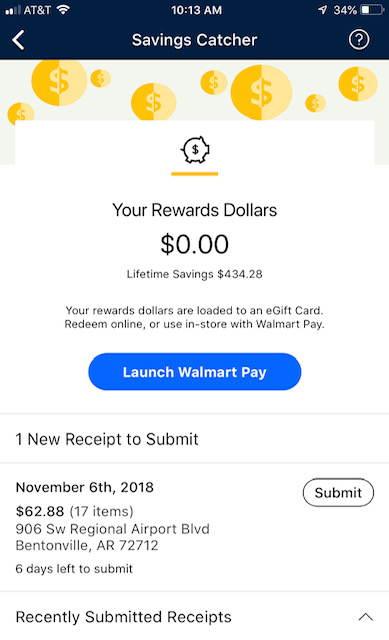This image is a screenshot of a cell phone displaying the Savings Catcher app. At the top, there's a dark blue bar with a white back arrow on the left and the app's name, "Savings Catcher," in white font centered. Below this bar, the wallpaper of the app features a pattern of eight coins, each with a dollar sign in the center. The coins are split into two color schemes: half light yellow and half dark yellow.

In the main window of the app, prominently displayed text reads "Your Rewards Dollars," showing a balance of "$0.00." Below that, it states "Lifetime Savings," displaying "$434.28." Further down, instructional text explains that "Your rewards dollars are loaded to any gift card. Redeem online or use in store with Walmart Pay." A blue button labeled "Launch Walmart Pay" is positioned beneath this text. At the bottom of the window, it indicates that there is "1 new receipt to submit."